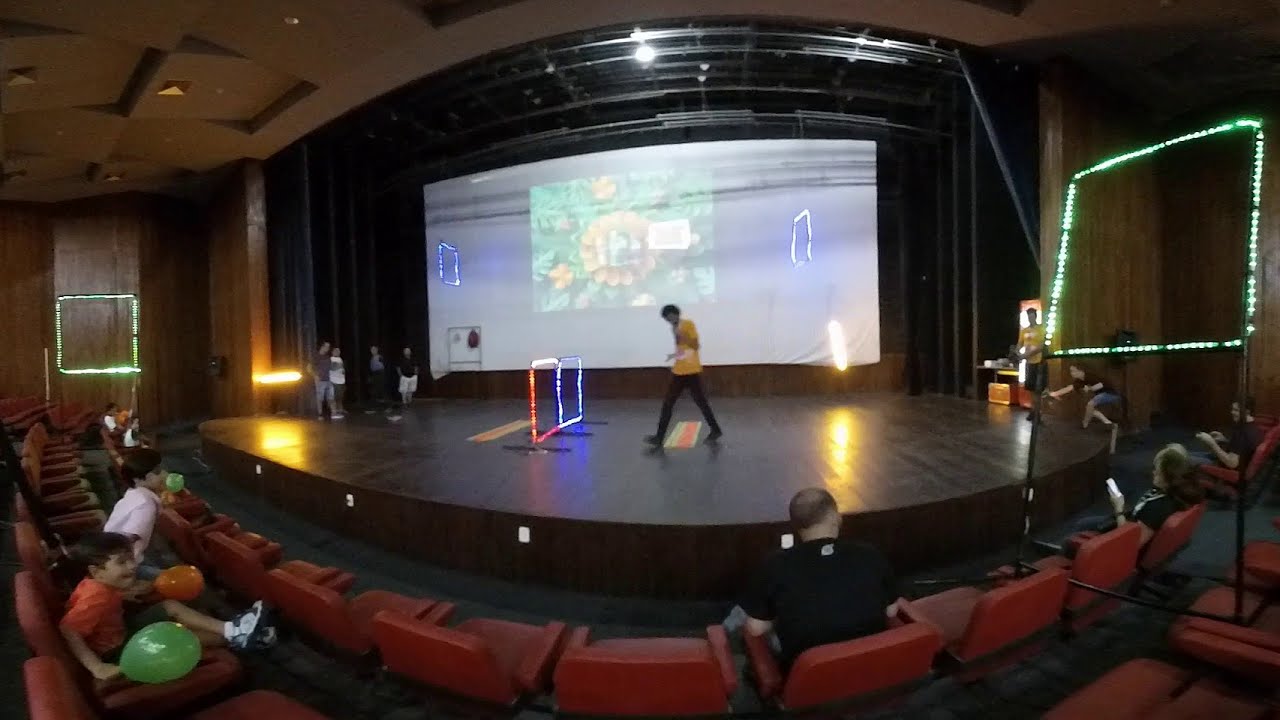In this vibrant, panoramic image captured inside a cozy theater, a slim man in a yellow shirt and black pants walks across a polished, raised wooden stage toward the center. The stage is adorned with two illuminated square frames—one outlined in red and white lights, and the other in blue and white lights. Behind the man, a massive projector screen displays a faint, colorful image of orange flowers against a green background, adding a picturesque flair to the setting. 

The theater seating consists of plush, red fold-up chairs typically found in movie theaters, with small lights lining the vertical portion of the stage. In the foreground, the audience comprises mostly small children, aged between six and nine, alongside a few adults. Notably, a child in the second row holds a green balloon in his right hand and an orange balloon in his left, with both legs up on the seat. 

There are adults standing on either side of the stage, some interacting with their smartphones. The scene has a unique fishbowl effect, bulging at the center and curving towards the edges, which accentuates the lively atmosphere and the colorful setup of this staged event.